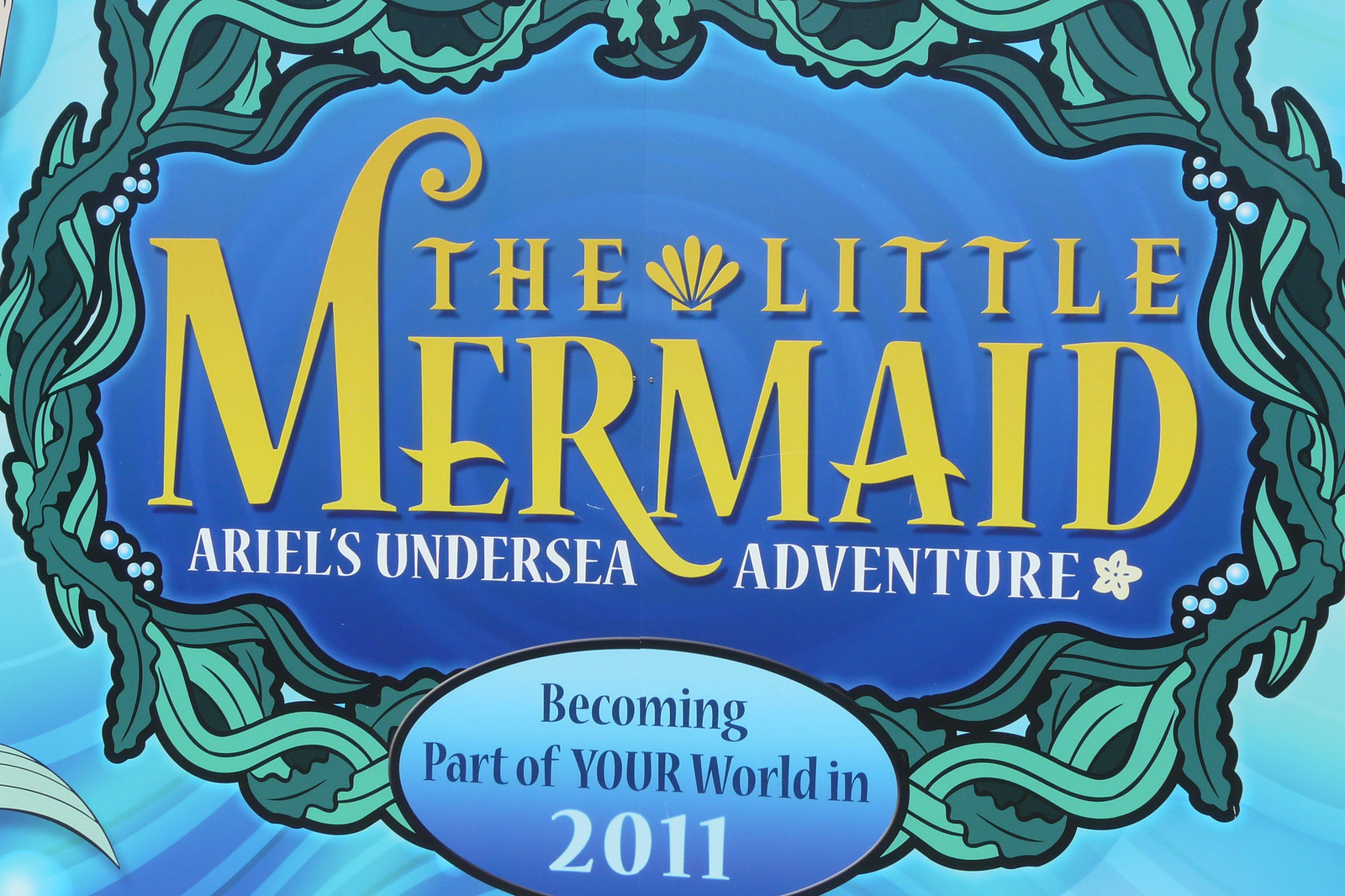This is a detailed advertisement for The Little Mermaid, showcasing a vibrant aquatic design. Dominating the center is the title "The Little Mermaid" in prominent yellow text. Directly beneath it, in smaller white text, it reads "Ariel's Undersea Adventure." The entire title is encased within an oval-shaped border of stylized green and blue seaweed, reflecting an underwater theme with hues of light and dark blue in the background. Adding to this, light blue scattered rays accentuate the aquatic atmosphere. In the middle of the seaweed oval, there’s a circular logo with an ombre effect transitioning from light to dark blue. This logo contains the phrase "Becoming Part of Your World in 2011" in blue text with the year 2011 highlighted in white. A subtle swirling pattern behind the title and delicate details like a white starfish enhance the overall whimsical undersea motif. This ad radiates the enchanting essence of The Little Mermaid's underwater world.